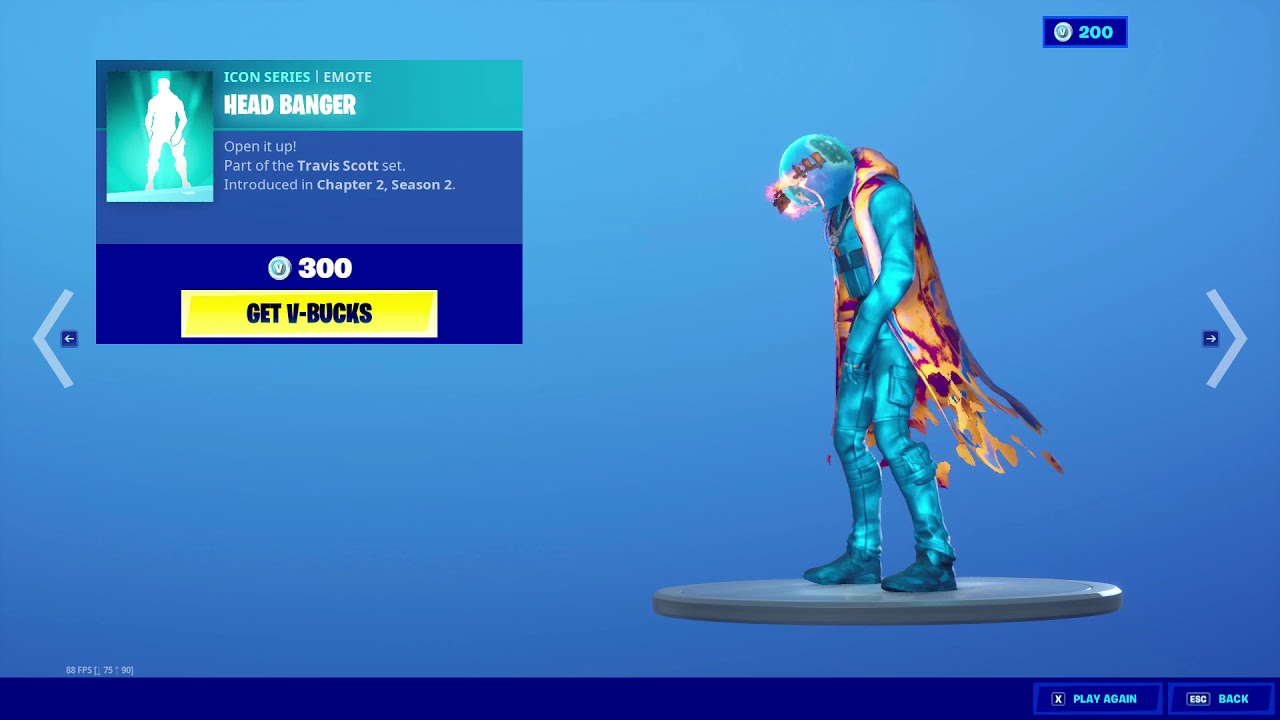The image appears to be a screenshot from a video game, likely Fortnite, indicated by the reference to V-Bucks. The overall background is a solid blue color, with a darker blue horizontal strip at the bottom, which serves as a border where light blue buttons labeled "Play Again" and "Back" are located. In the center-right of the image, a humanoid character with an alien-like appearance stands on a cement-gray round platform. This character is dressed in a blue suit, sporting a circular helmet and a gold, purple, and blue tattered cape that seems to be dripping pieces. The character is positioned against the solid blue background, giving a sense of prominence.

To the upper left of the image, there's a larger rectangular box that outlines a white character figure. To the right of this outline, the text reads "Icon Series, Emote, Headbanger" in bright white letters. Beneath this, it says "Open It Up, part of the Travis Scott set, introduced in Chapter 2, Season 2." Below this information is a number, "300," followed by a message "Get V-Bucks" on a yellow background. In the upper right-hand corner, another smaller rectangle displays the number "200," possibly indicating some form of score or currency in the game. 

Overall, the image seems to illustrate a character or item card from the game Fortnite, detailing a special emote and its associated set and purchase information.